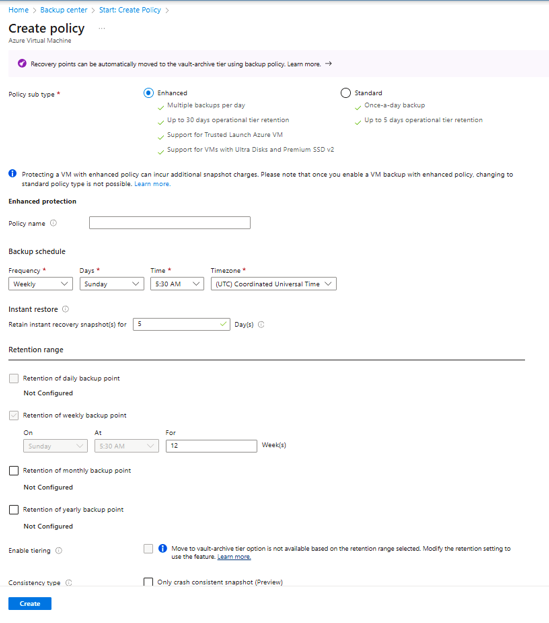The image appears to be a detailed screenshot of the "Create Policy" page within a desktop application or web platform, focusing on backup options for Azure Virtual Machines. In the top left corner, highlighted in blue text, are the labels "Home," "Backup Center," followed by "Start Create Policy," indicating the user is on a page where they can formulate a new backup policy. 

Below that, in bold, is the heading "Azure Virtual Machine," which signifies the backup applicability to Azure VMs. Under this heading is some informative text stating, "Recovery points can be automatically moved to the vault archive for using backup policy," accompanied by a blue hyperlink labeled "Learn more."

Next, a section labeled "Policy Subtypes" (marked with red asterisks to indicate importance) is visible. Two policy options are presented here. The first option, labeled "Enhanced," is selected by a blue radio button. Detailed benefits listed under this option, highlighted in green, include multiple backups per day, up to 30 days of operational tier retention, support for trusted launch Azure Virtual Machines, and support for VMs with Ultra Disks and Premium SSD version 2.

The second, non-selected option is labeled "Standard" and offers once-a-day backups with up to 5 days of operational tier retention.

The page is predominantly set against a white background, ensuring a clean and clear user interface.